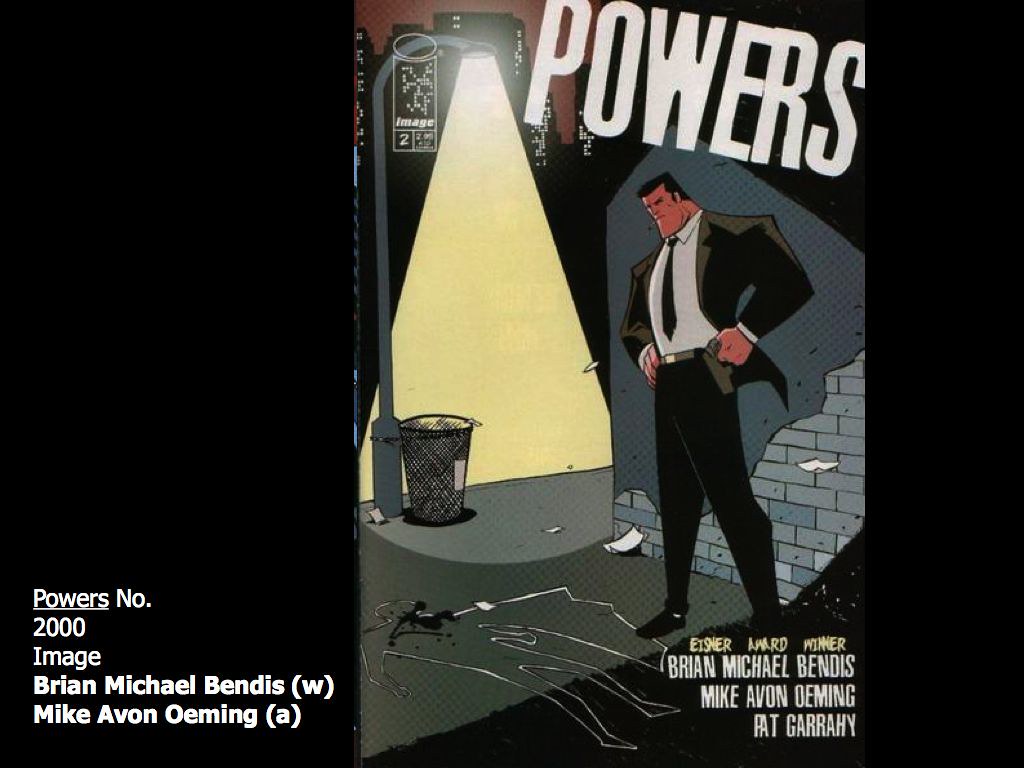The image appears to be a CD cover or a comic book cover predominantly featuring a scene in portrait orientation. In the bottom left corner, it reads "Powers," followed by "no," and then "2000," "Image," "Brian Michael Bendis (W)," and "Michael Avon Oeming (A)." Filling most of the frame is a comic book scene depicting a white man resembling Bruce Wayne; he wears a brown coat, black tie, and white shirt, and has a square head, broad shoulders, and a serious expression. He is standing in a dark back alley, illuminated by a streetlight, looking down at a chalk outline of a body with blood splatters around it. In the background, there's a trash can on the sidewalk, adding to the gritty atmosphere. The top right corner prominently features the word "Powers" in large white letters. In the bottom right, it states "Eisner Award Winner," followed by the names "Brian Michael Bendis," "Michael Avon Oeming," and "Pat Garrahay."